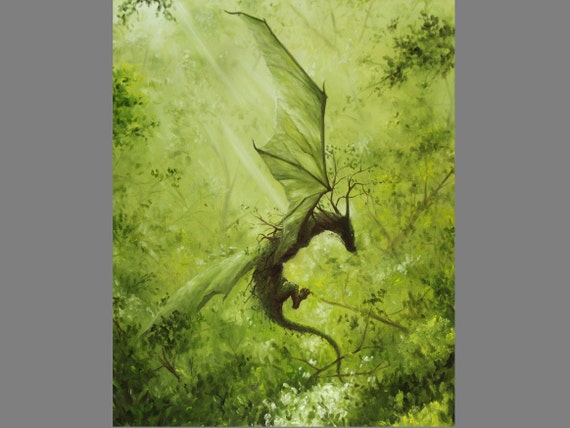The image features a dynamic, digitally rendered dragon with expansive, vibrant green wings, prominently positioned in the center. The dragon is depicted in mid-flight, viewed from a side angle, making it the focal point of the artwork. The background is rich with various shades of green, portraying lush trees and shrubbery, suggesting an outdoor daytime setting. The scene includes two green, square boxes and two rays of light. The combination of light and dark greens, accentuated with touches of black, white, and off-white, highlights the intricate detailing of the dragon and the surrounding foliage, emphasizing the creature's majestic presence against the natural backdrop.